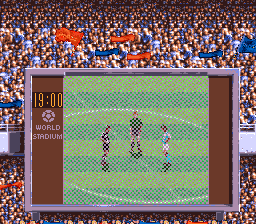The image appears to be a still from a computer-generated football game, reminiscent of visuals from the 1970s or 1980s. The central feature is a grainy screen displaying the center of the football pitch with the scoreboard indicating "19:00." The scoreboard is surrounded by a brown frame and the words "World Stadium" along with a soccer ball image. The field shows distinctive green stripes, common to classic football pitches, with an oval white section in the middle.

Within this oval, three pixelated figures are visible: the umpire, who wears an all-black uniform including shin guards, and two players. The player on the left is clad in a dark uniform, while the one on the right is in white or possibly light blue attire. Surrounding the field, a crowd is visible, holding various colored banners – some red, some blue, and a few orange. The spectators are indistinct, appearing as tiny dots in the distance, both above and below the central scoreboard.